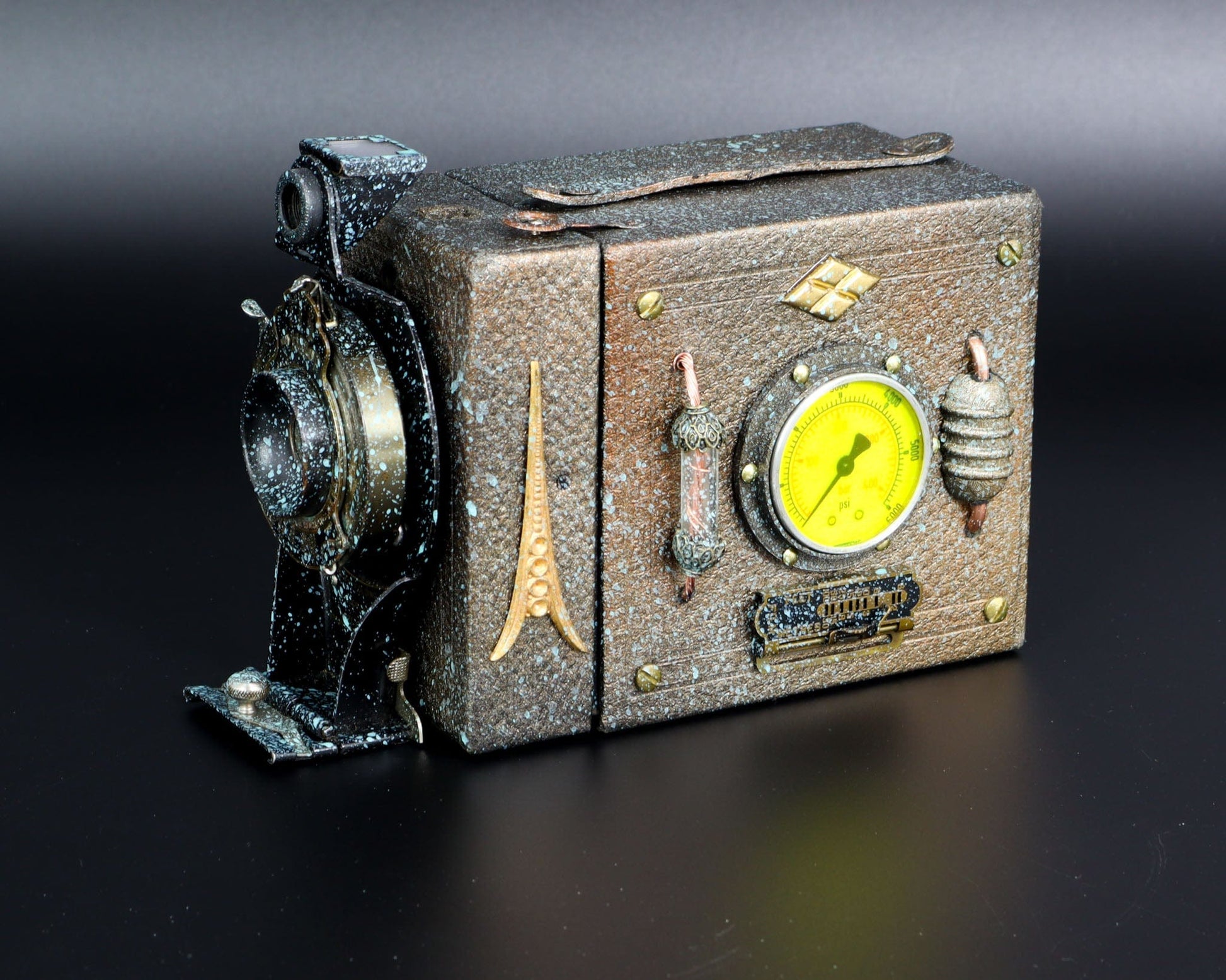This image showcases a vintage camera with a distinctive and detailed design. The camera appears to be made from metallic materials with a goldy-coppery hue, and it has accumulated green and white specks over time, suggestive of aging and use. The body of the camera is an elongated square shape, primarily dark brown. On the left side of the camera, there's a prominent black lens with white paint-like speckles, giving it a unique, weathered appearance. A notable feature on the side is a circular yellow meter or dial, which could be related to exposure settings, and has numbers around its edge with a single hand like a clock. The camera also has a black label on the front whose brand name is not entirely legible. Decorative bronze accents embellish the camera, including a gold piece resembling the Eiffel Tower on the front and additional gold decor in circle and diamond shapes on the right side. The front of the camera also showcases intricate designs, with some areas appearing hand-painted. A grip on the top indicates that the camera was designed to be portable. Overall, this camera merges functionality with ornate aesthetic details, making it a remarkable historic artifact.